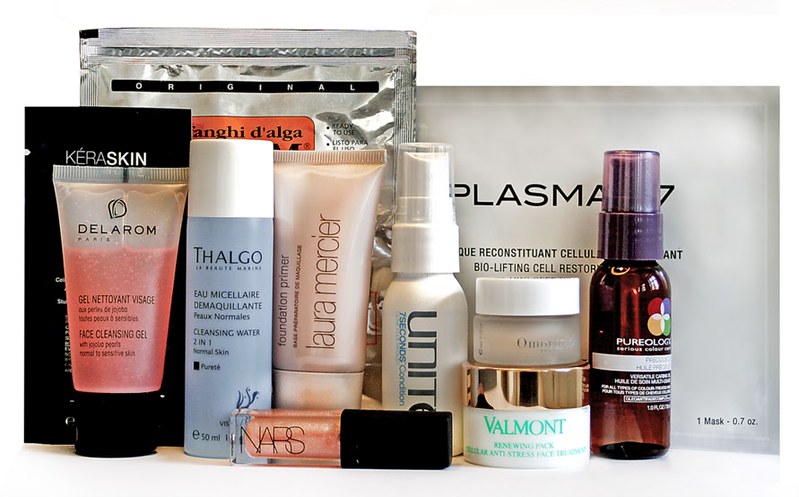A meticulously arranged lineup of various beauty products stands upright on a pristine white table against a clear, unobstructed background, likely intended for a product showcase image. 

Starting from the left:
1. A sleek black pouch emblazoned with the brand "Kera Skin" is partially obscured by another product.
2. In front of the pouch, a slender squeeze bottle identifies itself as "Deleram Face Cleansing Gel."
3. Behind this, a large silver pouch displays the word "Original" and features the brand "Fenghi Dialga." The product description is not visible.
4. Positioned in front of the silver pouch are four aligned products:
   - A light blue tube marked as "Thalgo Cleansing Water 2-in-1."
   - A "Laura Mercier" Foundation Primer.
   - An aerosol spray from "Unite" labeled as "Seven-Second Conditioner."
   - A small container, potentially lipstick, marked with the brand "NARS."

To the right and slightly behind this grouping:
1. A large white pouch with the discernible brand "Plasma" and a phrase that partly reads "Reconstitutent Cellular Bio-Lifting Cell Restoration."
2. Three products are arrayed before this pouch:
   - One small beauty container with an indistinct brand name, placed atop another container.
   - A product from the brand "Valmont," labeled as "Anti-Stress Face" with the remaining label unreadable.
   - An aerosol spray with the brand "Pureology," whose product details are also not visible.

This ensemble collectively conveys a sense of elegance and functionality across varied beauty essentials.